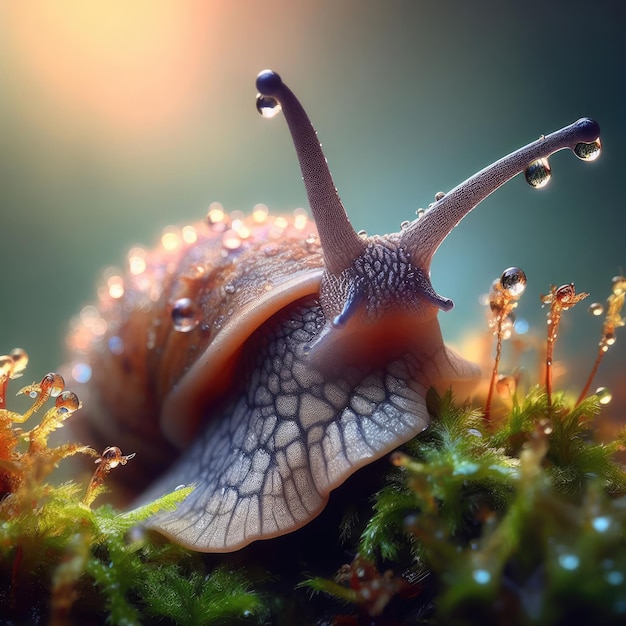This highly realistic 3D graphic image captures a close-up view of a snail in a natural outdoor setting, possibly after rainfall or early in the morning due to the visible dew. The snail, with a light beige body marked by black vein-like lines giving it a scaly appearance, has two prominent purple-tinted antennas with droplets at their tips. The shell, light brown and speckled with moisture, contrasts with the vivid green moss or grass below, which also glistens with dew. In the bottom right corner, a green plant further emphasizes the lush and wet environment. The background, a blend of green with hints of blue, adds depth to the scene, enhancing the overall realism of the image.